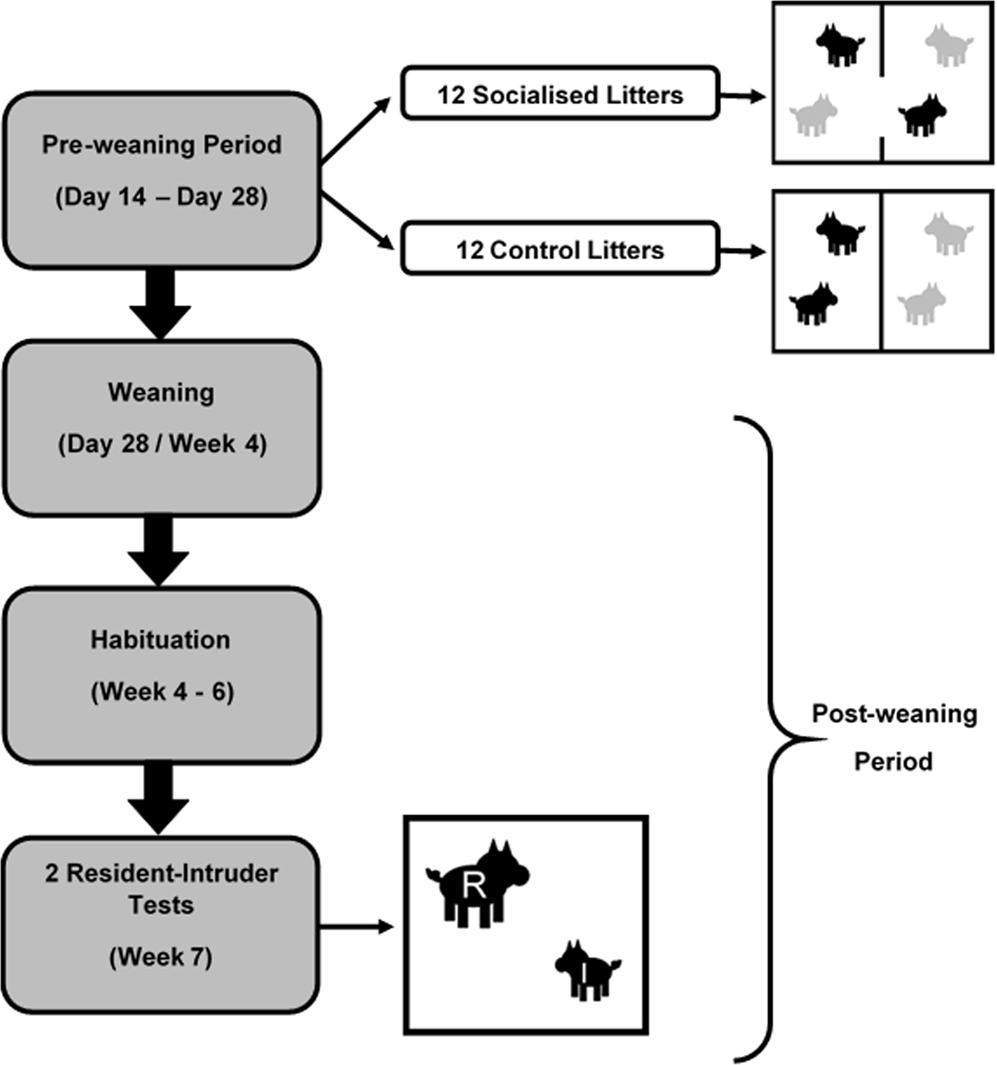This vertical image features a detailed flowchart illustrating the developmental stages of puppies, particularly focusing on their weaning periods and socialization. Starting on the left, there are four main boxes with dark backgrounds and black text. The first box labeled "Pre-Weaning Period" spans from day 14 to day 28. Below it, an arrow points to the second box, "Weaning," which covers from day 28 to week 4. The third box, "Habituation," ranges from weeks 4 to 6, and the fourth box represents "Two Resident Intruder Tests" conducted during week 7.

Branching off from the "Pre-Weaning Period" box, two pathways emerge. One pathway leads to "12 Socialized Litters," depicted with a box featuring four dogs—two black and two gray—freely moving between open lines. The other pathway leads to "12 Control Litters," shown with two black dogs and two gray dogs separated into smaller, confined areas.

Continuing down, the flowchart transitions to a final segment showing silhouettes of a larger dog marked with an 'R' and a smaller dog marked with an 'I,' signifying the "Post-Weaning Period." This comprehensive flowchart combines each caption’s insights to provide an extremely detailed representation of the puppies' developmental stages and their socialization status.